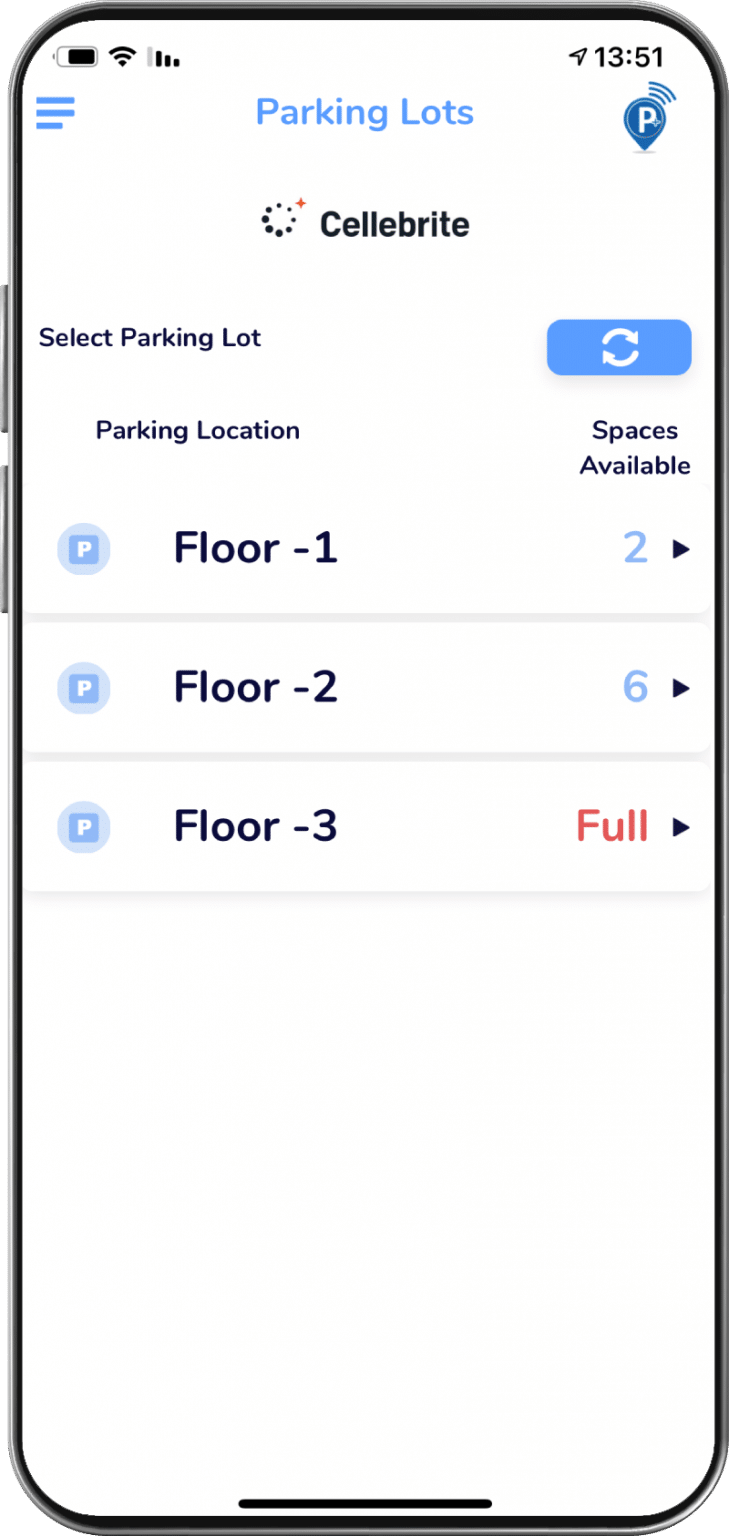A person is using their smartphone to locate available parking spaces. The time displayed is 13:51, and the phone shows a nearly full battery (around 7/8ths) with a strong network connection. They have searched for parking lots and the first result is "Sell Bright." Upon selecting this parking lot, the app presents a user-friendly interface featuring a blue button with two half-circle arrows indicating refresh capabilities. 

The app provides detailed information about parking availability across different floors. On the first floor, there are 2 available spaces; on the second floor, there are 6 available spaces; the third floor, however, is marked completely full with the word "full" highlighted in red. This feature helps users decide their parking strategy before even arriving at the garage. The app is useful for checking multiple parking garages, ensuring users can easily find and select the best parking options based on real-time availability.